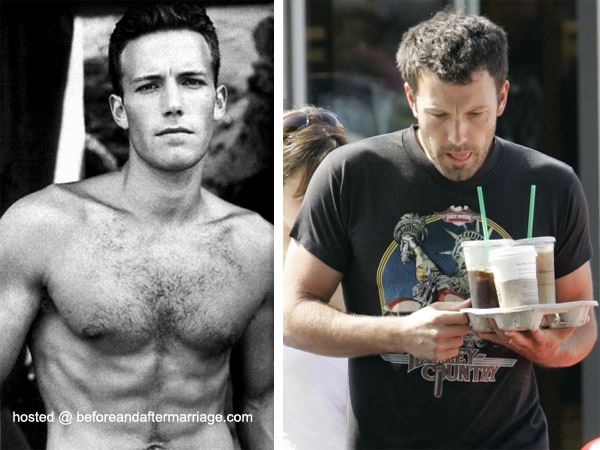The image features a split view of Ben Affleck, serving as a "before and after" portrayal, presumably related to marriage, as indicated by the watermark from beforeandaftermarriage.com. The left side of the image is a black and white photograph of Affleck in his younger years, topless and modeling. He has short, spiked brown hair, is clean-shaven, and displays a fit yet slender physique, with visible abs. The right side presents a candid shot of Affleck more recently, dressed casually in a black t-shirt, holding a tray with three coffees—two with green straws and one white cup—while looking down at them. He appears slightly disheveled with some scruff on his face, suggesting he might have just woken up for a coffee run. This detailed juxtaposition underscores the contrast between his younger, refined appearance and his current, more relaxed demeanor.